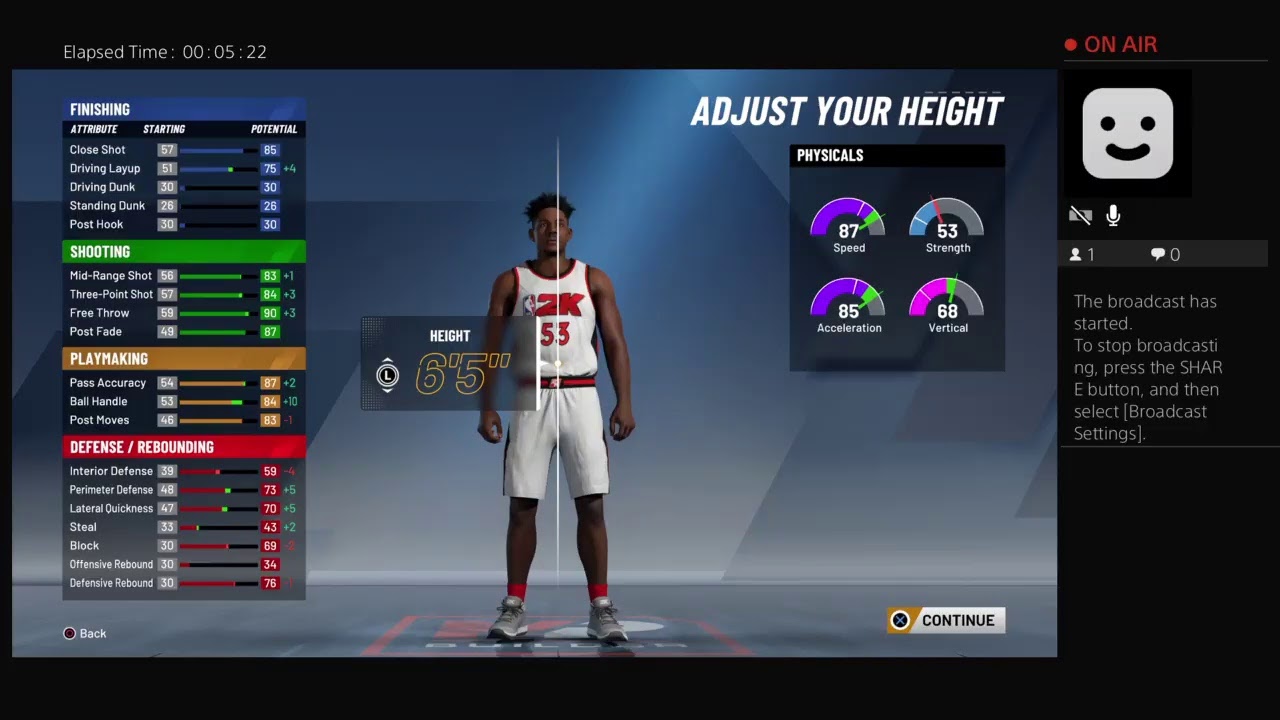The image is a screen capture from an online application, showcasing a 3D simulation of a man standing. The man is depicted wearing a white basketball jersey and matching shorts, complemented by grey sneakers. He sports a short afro hairstyle. On the left side of the simulation, in large text, the height of the man is indicated as 6 feet 5 inches. The screen features a black frame or border, and the primary background for the simulated figure is a greyish-blue color.

To the left of the simulated man are various statistics presented in white text, accompanied by colorful bars in blue, green, orange, and red. On the right side of the screen, in large white font, the words "Adjust Your Height" are prominently displayed.